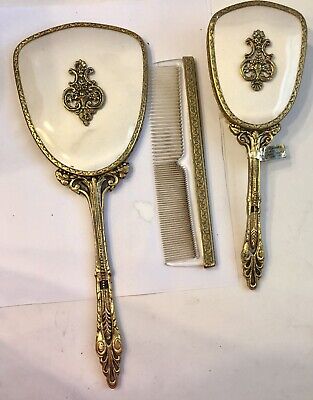The image depicts a vintage grooming set consisting of three pieces: a large hand mirror on the left, a comb in the middle, and a smaller hairbrush on the right. These items are positioned on a white surface, potentially on top of a white piece of paper, and are shown from the back. Each piece is adorned with ornate, tarnished silver detailing, suggesting they are made of silver or a similar metal.

The back of both the hand mirror and the hairbrush features a mother-of-pearl or porcelain-like material with a central, intricate silver crest or emblem which is somewhat obscure due to the detailed scrollwork. The long, narrow handles of the mirror and brush exhibit elaborate, possibly Victorian or Edwardian-era designs with swirling patterns and textures, indicative of their antique nature.

The comb, situated centrally between the mirror and brush, has fine metal teeth with an ornate silver back, showing signs of age and wear. The entire set, bathed in light from an unspecified source creating shadows to the lower left, exudes a sense of historical elegance and meticulous craftsmanship.